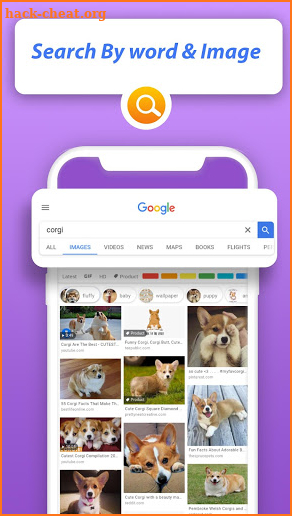The image displays a vibrant purple background framed by an orange rectangular border. At the top center, the text "back-cheat.org" is written in bold orange letters. Below this, a curved-edge rectangle contains the words "search by word and image," also in orange. Further down, there is a white magnifying glass icon encased in an orange circle.

Towards the bottom of the image, a white smartphone is depicted with a Google search interface visible on its screen. The search term entered is "corgi." Displayed on the phone are a series of thumbnail images of corgis. On the left side of the screen, there are four pictures of corgis. In the middle section, there are two corgi images, and on the right side, there are three corgi pictures. The various images show both single and multiple corgis, ranging from puppies to adult dogs, all of which are irresistibly cute.